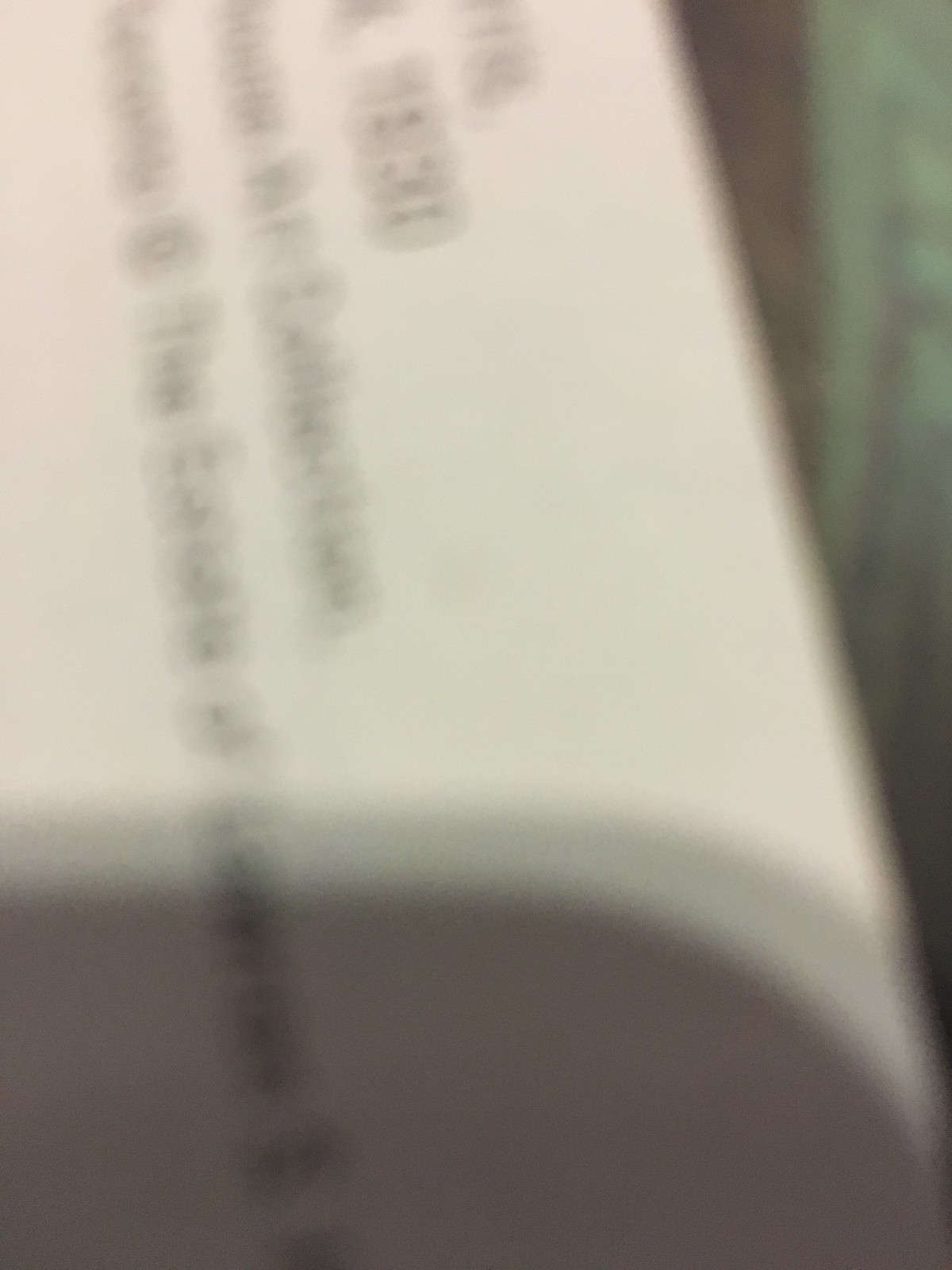A blurry, vertical photograph taken indoors features an image of a white paper with black, unreadable text. The photograph appears to have been rotated, causing the text to run vertically down the image instead of the conventional horizontal orientation. In the background, there is a narrow strip of darkness and a small patch of green, possibly indicating nearby objects or furniture. The bottom fourth of the photo is obscured by a shadow cast by the cell phone used to capture the image, adding to the overall lack of clarity.